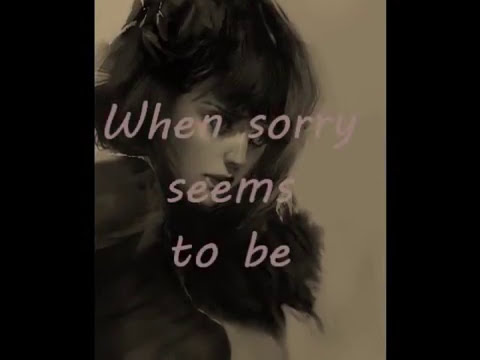The image features a light cream-colored background with two vertical black bars on the left and right sides. In the center, light purple text reads "when sorry seems to be." The text partially obscures a detailed sketch of a woman with a serious expression. She is offset to the left, staring to the right, with large eyes and prominent whites, and her hair styled in a bob reaching her neck. She is dressed in a snug, dark-colored shirt. The woman's face and upper body are visible, though some features are masked by the text.